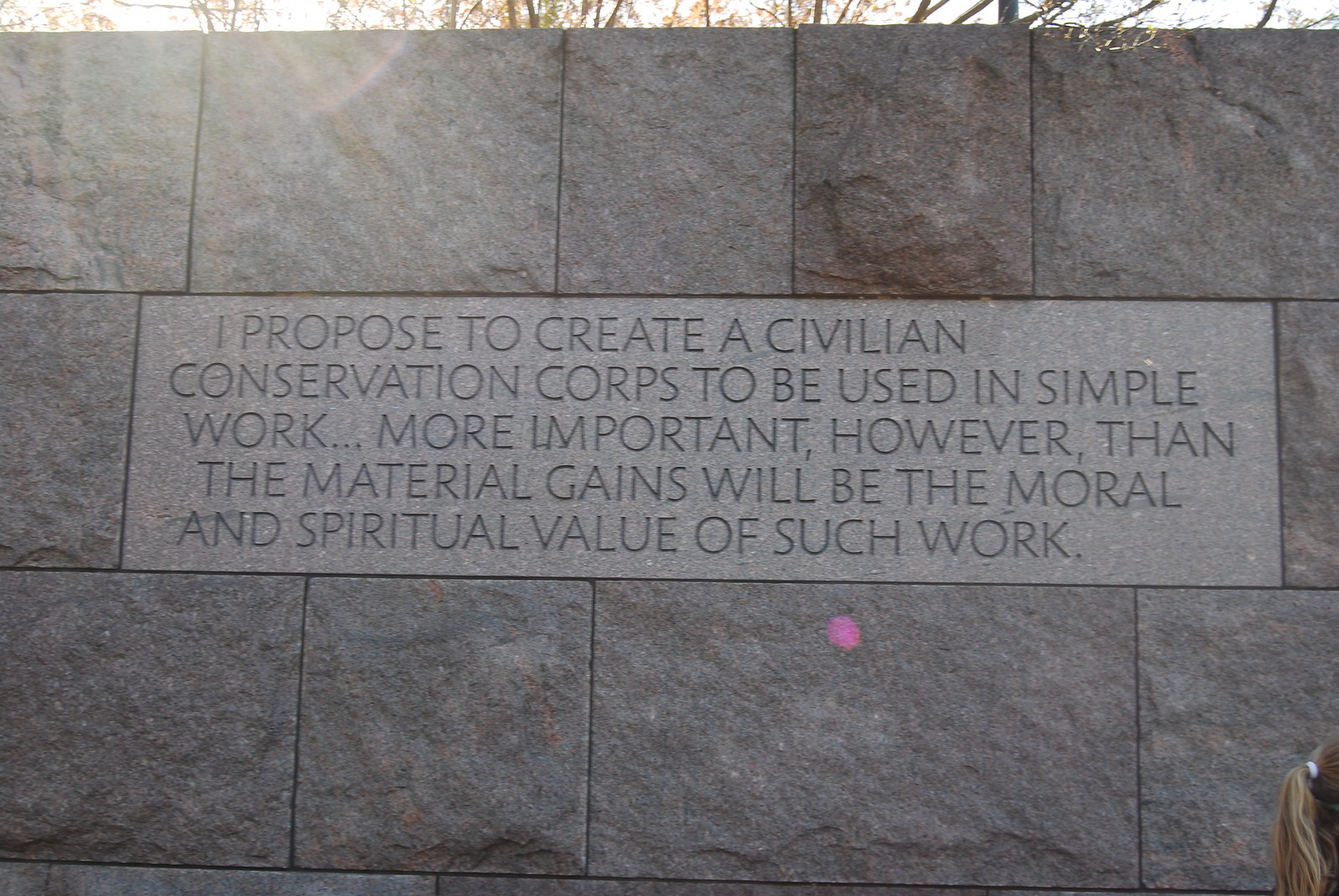The photo, taken outdoors in bright sunlight, showcases a predominantly stone wall composed of variously sized rectangular and square bricks. The bright sun rays create a noticeable glare, particularly in the top left, and cause occasional lens flares, including a pink dot in the lower portion of the wall. Centered on the smoother surface of the wall is an engraved plaque bearing the inscription: "I propose to create a civilian conservation corps to be used in simple work. More important, however, than the material gains will be the moral and spiritual value of such work." The image also captures the top of some trees with yellow leaves, indicating autumn, and a small section of a girl's blonde ponytail in the lower right corner.